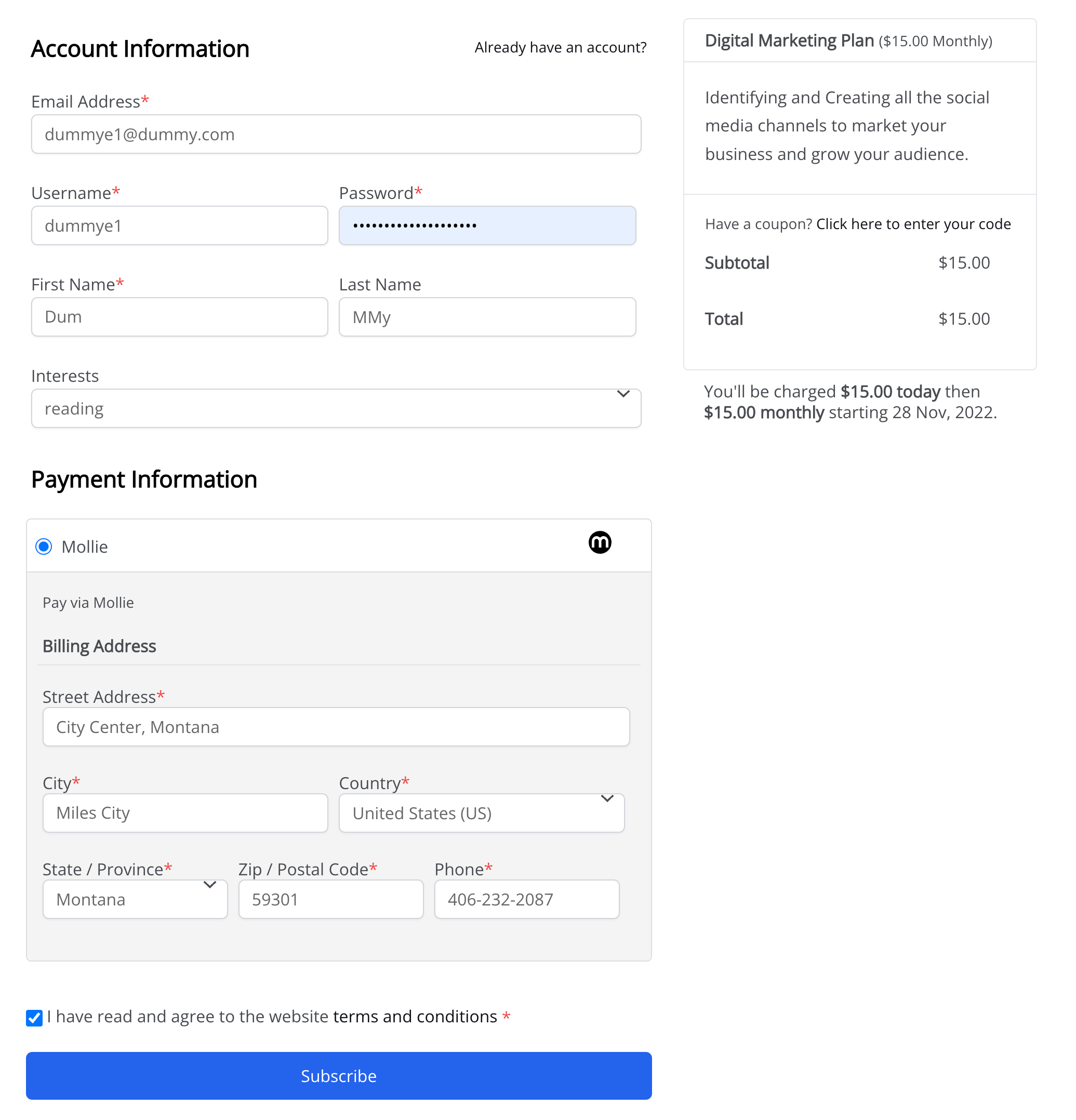The image displays a form for account registration and payment on the left side, accompanied by a summary of a digital marketing plan on the right.

**Left Side:**
- **Account Information:**
  - **Email Address:** Labeled with black text, followed by a red asterisk (*), indicating a required field. The placeholder text in the input bar is "dummy1@dummy.com."
  - **Username:** Also marked with a red asterisk (*), with the username input as "dummy1."
  - **Password:** Accompanied by a red asterisk (*), with the field obscured by approximately 12 black dots representing hidden characters.
  - **First Name:** Entered as "dum."
  - **Last Name:** Entered as "mmy."
  - **Interests:** Listed as "reading."

- **Payment Information:**
  - **Mobile Payment Option:** Indicated by bold black text with a blue circle icon.
  - **Billing Address:**
    - **Street Address:** Listed as "city center Montana."
    - **City:** Entered as "mile city."
    - **Country:** "United States."
  - At the very bottom, there is a blue bar containing the "Subscribe" button.

**Right Side:**
- **Digital Marketing Plan:**
  - Subscription details are presented at the top with the text: "Digital Marketing Plan ($15 monthly)."
  - Below this, a description reads: "Identifying and creating all the social media channels to market your business and grow your audience."
  - Pricing details are provided:
    - **Subtotal:** $15
    - **Total:** $15
    - A final note indicates, "You'll be charged $15 today, then $15 monthly starting 28th November 2022."